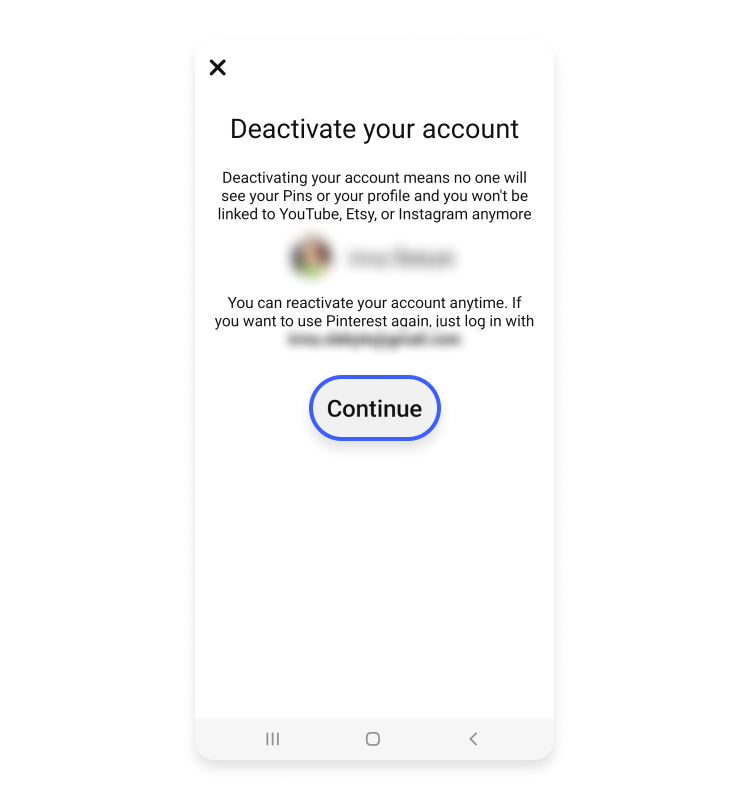The image depicts a mobile pop-up notification with a white background, resembling a deactivation confirmation screen. At the top left corner, there is a black 'X' icon, symbolizing the option to close the pop-up. The headline "Deactivate your account" is prominently displayed in bold black text. Below the headline, a detailed message informs the user that deactivating the account will hide their pins and profile and sever links to YouTube, Etsy, and Instagram.

A profile picture featuring a person's image is visible. The design includes a darker hue on the left, transitioning to a reddish color on the right, with a lime green bottom section. The name or identifier beneath the profile picture is obscured by white.

Further down, the message assures users that they can reactivate their account at any time by logging in, noting this detail in non-legible black text grayed out for emphasis. At the bottom of the pop-up, a blue-outlined, gray 'Continue' button stands out, with "Continue" written in bold black letters inviting users to proceed. The image captures the entire notification, clearly indicating it is from a mobile device, as denoted by the visible device icons at the bottom.